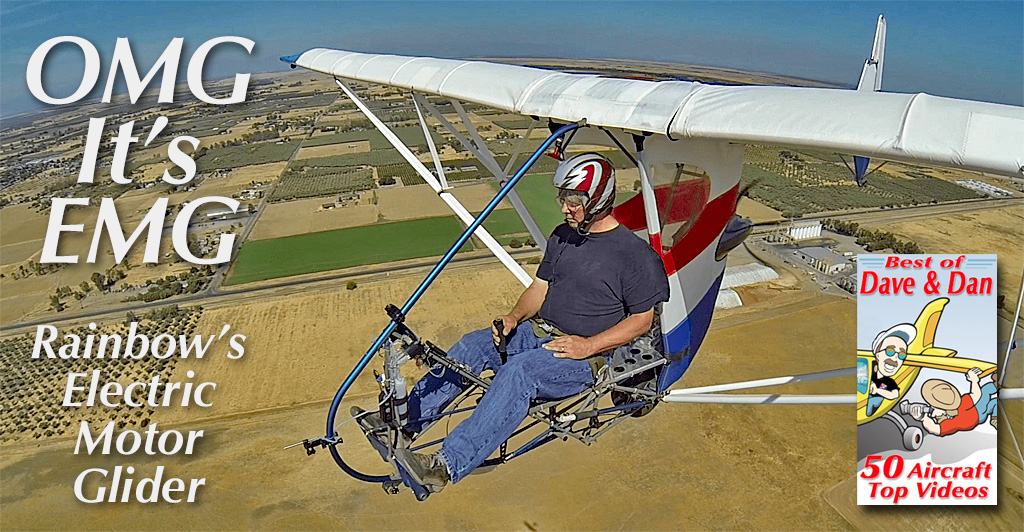The photograph shows an advertisement with prominent large white text on the top left reading "OMG it's EMG," and slightly smaller white text below it stating "Rainbow's Electric Motor Glider." In the bottom right corner, there is a red-labeled image of a book titled "Best of Dave and Dan" with a subtitle of "50 Aircraft Top Videos." The main focus of the image is a man flying in a single-seat electric motor glider. He is wearing a silver and red helmet with a black strap, a short-sleeved black shirt, blue jeans, and brown shoes. The glider, which has large white wings and a frame with white supports tied by a blue structure, features a body painted in white, red, and blue behind the pilot. The man, seated with his hands on a control stick or lever, is flying high above a landscape comprising green and yellow rectangular plots of farmland, with a sky above that is mostly white, revealing some distant gray clouds near the horizon.